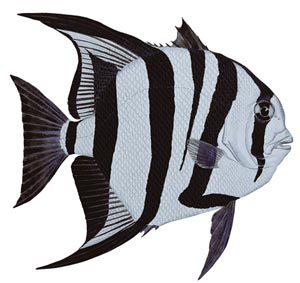This image is a detailed and realistic side profile illustration of a fish, resembling a zebrafish or angelfish, depicted in black and white. The fish faces to the right with a completely white background. It features an off-white body adorned with five prominent black stripes including one that runs vertically through its eye. The eye is black and quite noticeable, and the small mouth appears slightly open. The fins are distinct and varied: a small black dorsal fin on top, a larger striped fin extending from its mid-back, and a fan-like tail fin mostly black but highlighted with subtle white accents. Additionally, there's a small, dark gray fin positioned towards the front bottom, and a light, see-through gray fin located in the middle of the body. Despite the monochrome palette, the fish's detailed scales and stripe patterns create a vibrant and textured appearance.